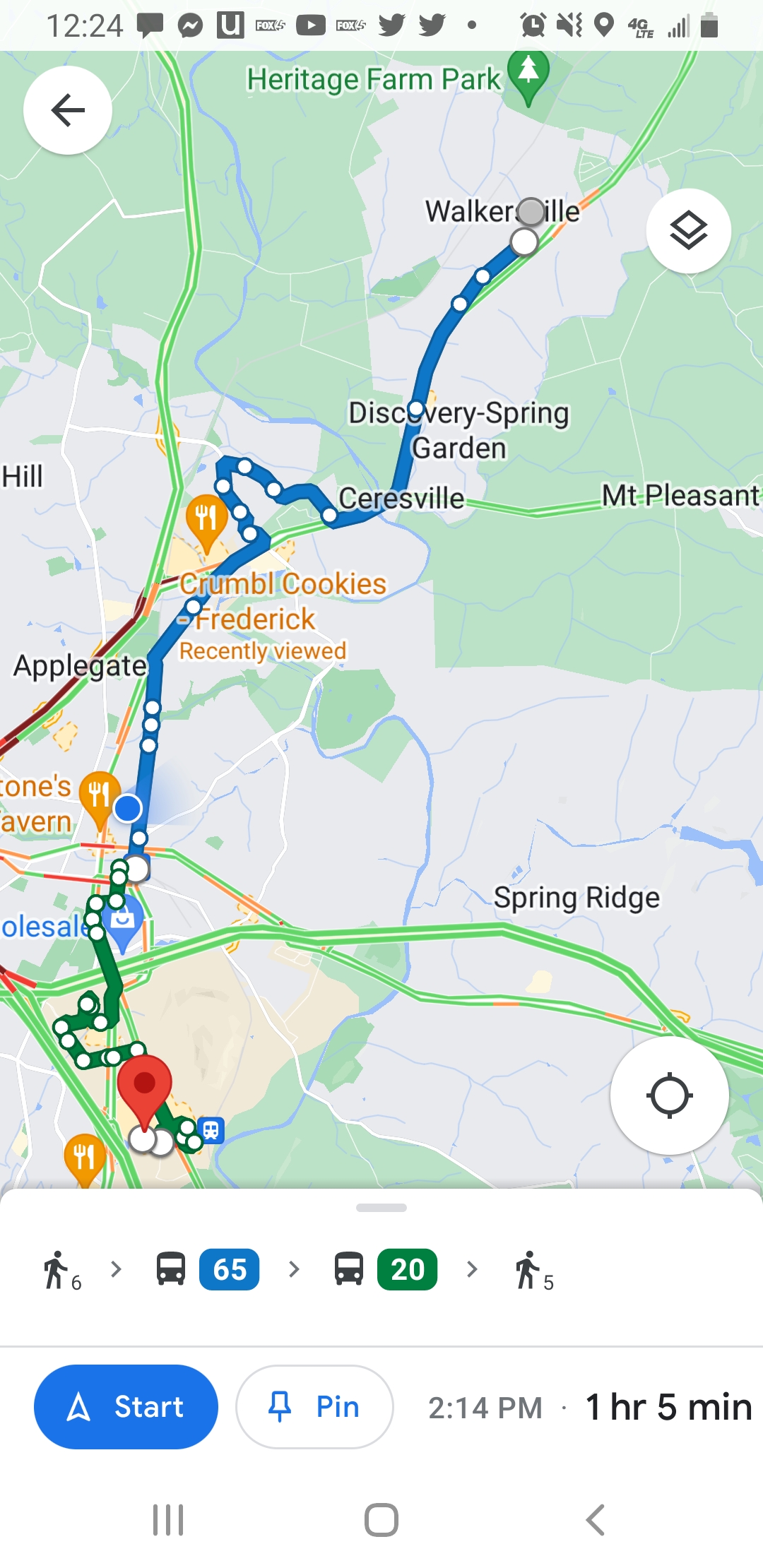This image depicts a digital map interface, similar to one you might find on a smartphone. The map is centered on an area labeled "Spring Ridge" and includes notable points such as "Crumble Cookies Frederick," "Applegate," "Mount Pleasant," and "Discovery Spring Garden." A highlighted route is visible, beginning with a green line that transitions into a blue line, indicating the path from point A to point B. The route originates from the lower part of the map, marked by a red teardrop icon, and is mapped out as a 1-hour and 5-minute walking distance. The map's background suggests that the surrounding area is predominantly green, hinting at lush, natural scenery.